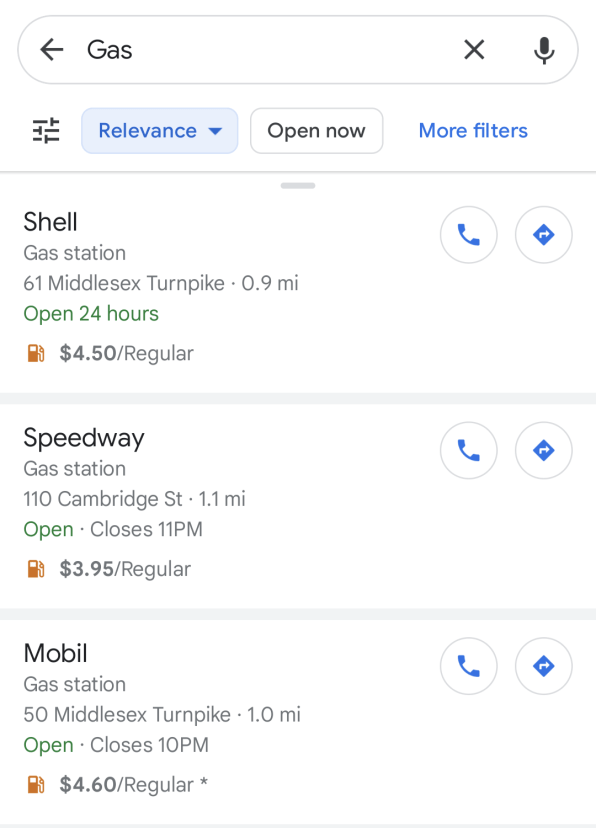This screenshot depicts a search results page for gas stations, taken in portrait mode with a white background. The layout is structured in a single column. 

At the top, there's a search bar featuring a back arrow on the left, followed by the search query "gas" which the user has entered. On the right side of the search bar, there are two icons: an 'X' for clearing the search and a microphone for voice input.

Below the search bar are filter options. The first icon is for filters, followed by a blue button labeled "Relevance" with a downward arrow indicating that the results are sorted by relevance. Next is a button labeled "Clear," which is associated with an option that says "Open Now." The last tab in this row is in blue and labeled "More Filters."

The search results are presented in three rows:

1. **Row 1:**
   - **Gas Station:** Shell
   - **Address:** 61 Middlesex Turnpike
   - **Operating Hours:** Open 24 hours (shown in green)
   - **Price:** $4.50 for regular gas
   - On the right side, there are two icons: a call button and a diamond with a right arrow, possibly for more details or to visit the gas station's webpage.

2. **Row 2:**
   - **Gas Station:** Speedway
   - **Address:** 110 Cambridge Street
   - **Operating Hours:** Open now, closes at 11 PM
   - **Price:** $3.95 for regular gas
   - Similar to the first row, it features a call button and a diamond with a right arrow on the right side.

3. **Row 3:**
   - **Gas Station:** Mobile
   - **Address:** 50 Middlesex Turnpike
   - **Operating Hours:** Open now, closes at 10 PM
   - **Price:** $4.60 for regular gas
   - This row also includes a call button and a diamond with a right arrow on the right side.

Overall, the image serves as a filtered search result page, providing detailed information about gas stations, including their locations, prices, and operating hours.